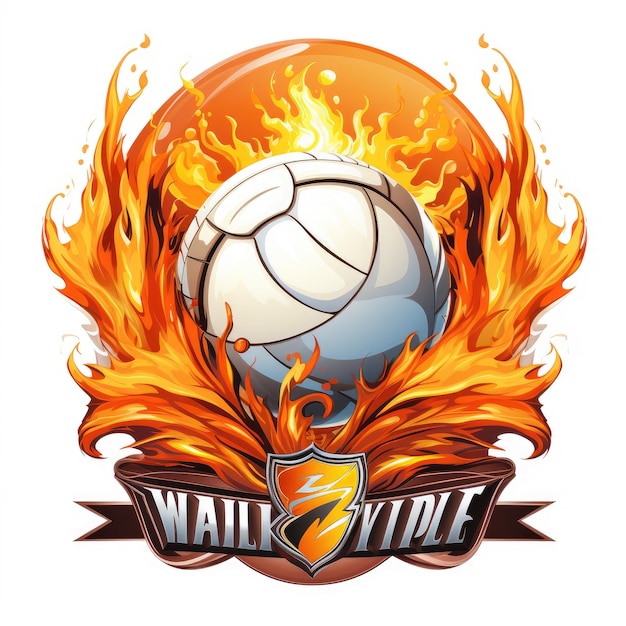This color illustration, set in a square format, depicts a dynamic and fiery team symbol. At the center, there is a white ball, possibly representing a soccer or volleyball, adorned with circular lines and brown patterns. This ball is engulfed in vivid orange and yellow flames that extend dramatically to the left and right, creating an elliptical shape, and are mirrored by similar flames in the background. Behind the flaming ball, there's an orange circular pattern adding depth and intensity to the scene. Prominently in the foreground, a dark brown banner with notched ends spans the lower portion of the image, emblazoned with the text "WAILIBIPLE" in white letters. Overlapping this banner is a yellow and orange logo, shaped like a seal, featuring a central shield with black and white arrowed swirls against a gradient background. The entire scene is set against a white backdrop, highlighting the vivid colors and intricate details of the fiery emblem.